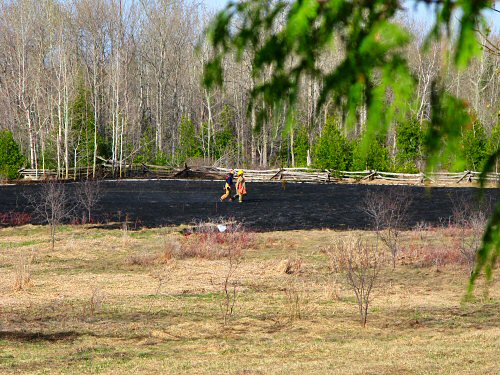In this outdoor photograph, two small figures, potentially children or people wearing yellow hats, are seen walking in the distance across a field. One figure appears to be donning a dress, while the other is possibly dressed in a blue shirt and khakis. The foreground features a stretch of dead grass, scattered thin twigs, and dead weeds, with a tree branch overhanging from the top right corner, slightly out of focus. The ground behind the figures is notably dark or black, suggesting a recent controlled burn or forest fire, yet the surrounding areas remain unaffected. These figures are casting shadows as they walk towards a simple wooden split rail fence, consisting of long wooden bars which demarcate the edge of the field. Beyond the fence lies a forest backdrop comprising green pine trees, alongside numerous tall, leafless trees with white stems, indicative of the changing seasons. A large shadow stretches out in front of the fence, engulfing the area where the two figures are located. The scene is capped by a clear blue sky.